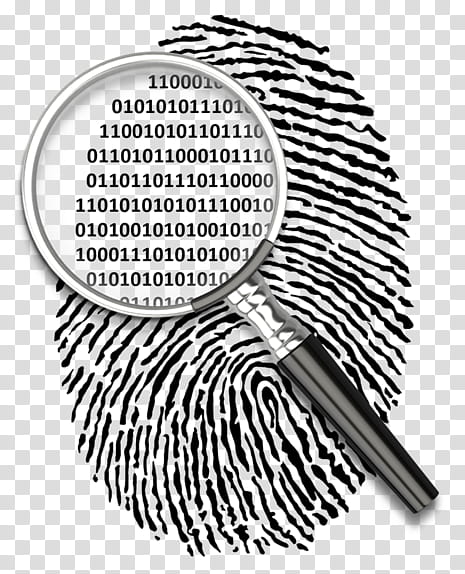The image is a detailed black and white illustration with a grey and white checkered background, resembling the transparency grid of a PNG file. At the center is a large black fingerprint, where the negative spaces between the black lines reveal the checkered background. Diagonally spanning from the lower-right corner to the upper-left corner is a magnifying glass with a black handle and a metallic attachment connecting the handle to the glass. The glass portion of the magnifying glass features a silver metallic rim. Through the magnifying glass, a section of the fingerprint is magnified, and within this section, the lines of the fingerprint are replaced by a series of binary code, composed of ones and zeros, seamlessly following the fingerprint’s pattern. The entire image is vertically oriented and composed to emphasize the interplay between the fingerprint and digital data.